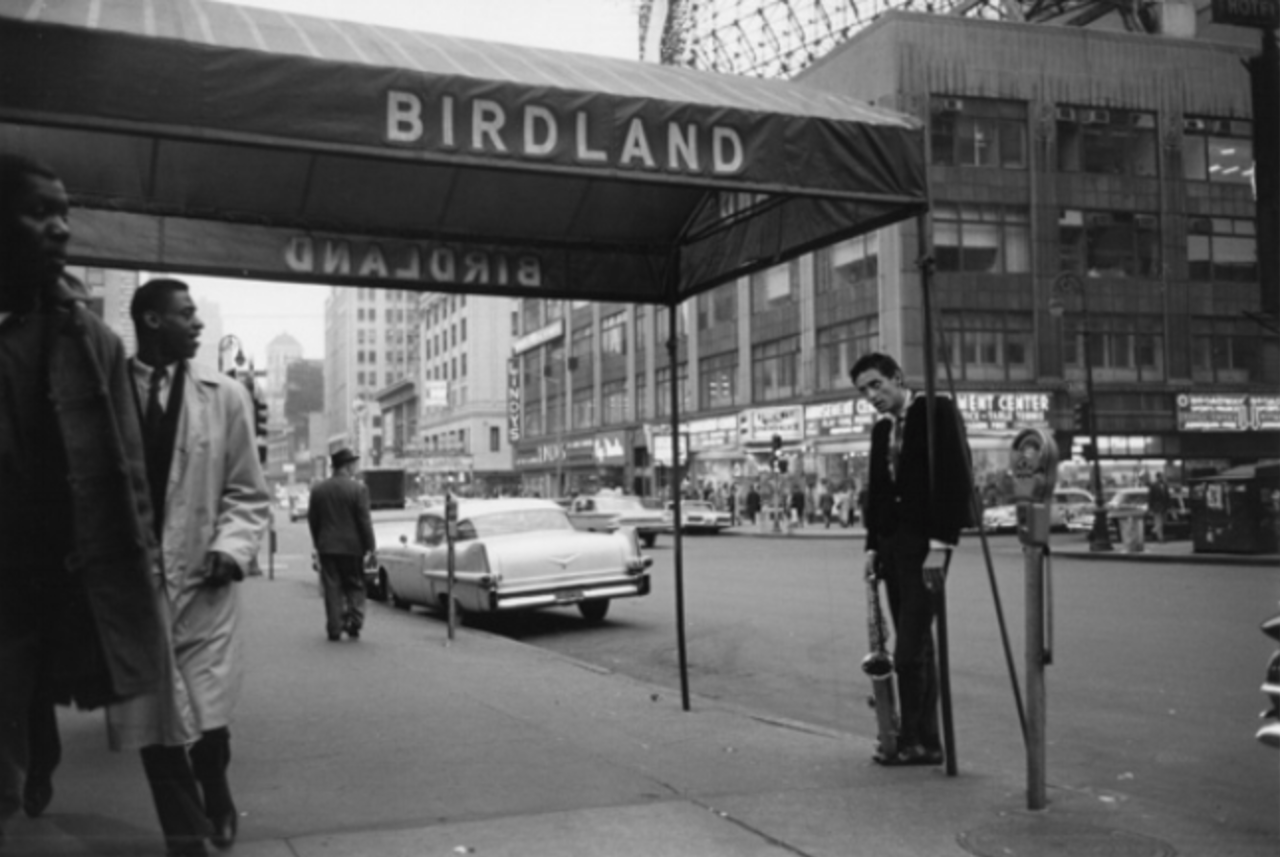In this detailed black-and-white photograph taken in New York City during the late 1950s to mid-1960s, the iconic Birdland Jazz Club sign hangs prominently above the sidewalk. A white car, indicative of the 1960s or 1970s style, is parked nearby. The scene centers around a white musician leaning with a saxophone resting on his foot, possibly taking a break from playing. This saxophonist stands beside a parking meter and is situated under the Birdland canopy, which extends outward from the club's entrance supported by two poles. To the far left of the image, two African-American men in coats—one in a trench coat and the other in a shorter coat—are either walking by or entering the club. They appear to be either observing the musician or something beyond him. Across the street is a three-story building with numerous windows, part of a shopping center that attracts several pedestrians, although the street seems relatively free of heavy traffic. Further down the sidewalk, a lone man walks in the distance, enhancing the nostalgic cityscape captured in this vintage urban setting.